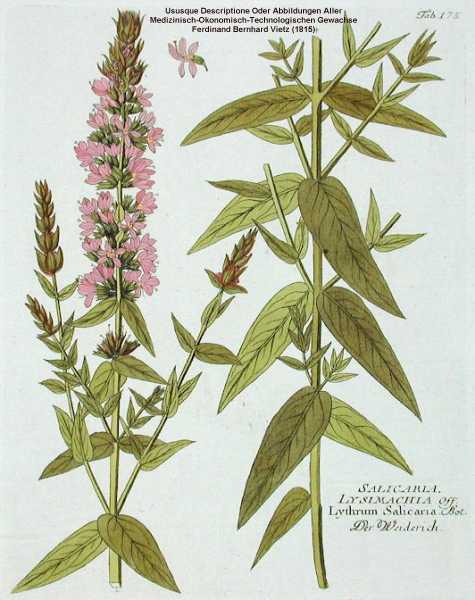The image portrays a detailed botanical illustration of two plants. On the left, the plant features delicate pink flowers sprouting from a green stem, with long and thin light green leaves that get progressively narrower towards the center of the drawing. To the right, the plant is characterized by larger green leaves without any flowers, suggesting it might be a different stage or part of the same species. Suspended between the two plants, near the top of the image, is a singular pink flower in mid-bloom. The top right corner of the image is labeled "FAB-175," and the bottom right corner includes text in a foreign language: “SELICAROLE LACIMARTIER LITHIUM SELICARIA DR. WONDERWICK.” This detailed illustration, with its descriptive labels and focus on different parts of the plant, likely originates from a botanical textbook or brochure, aimed at categorizing and studying this particular species.